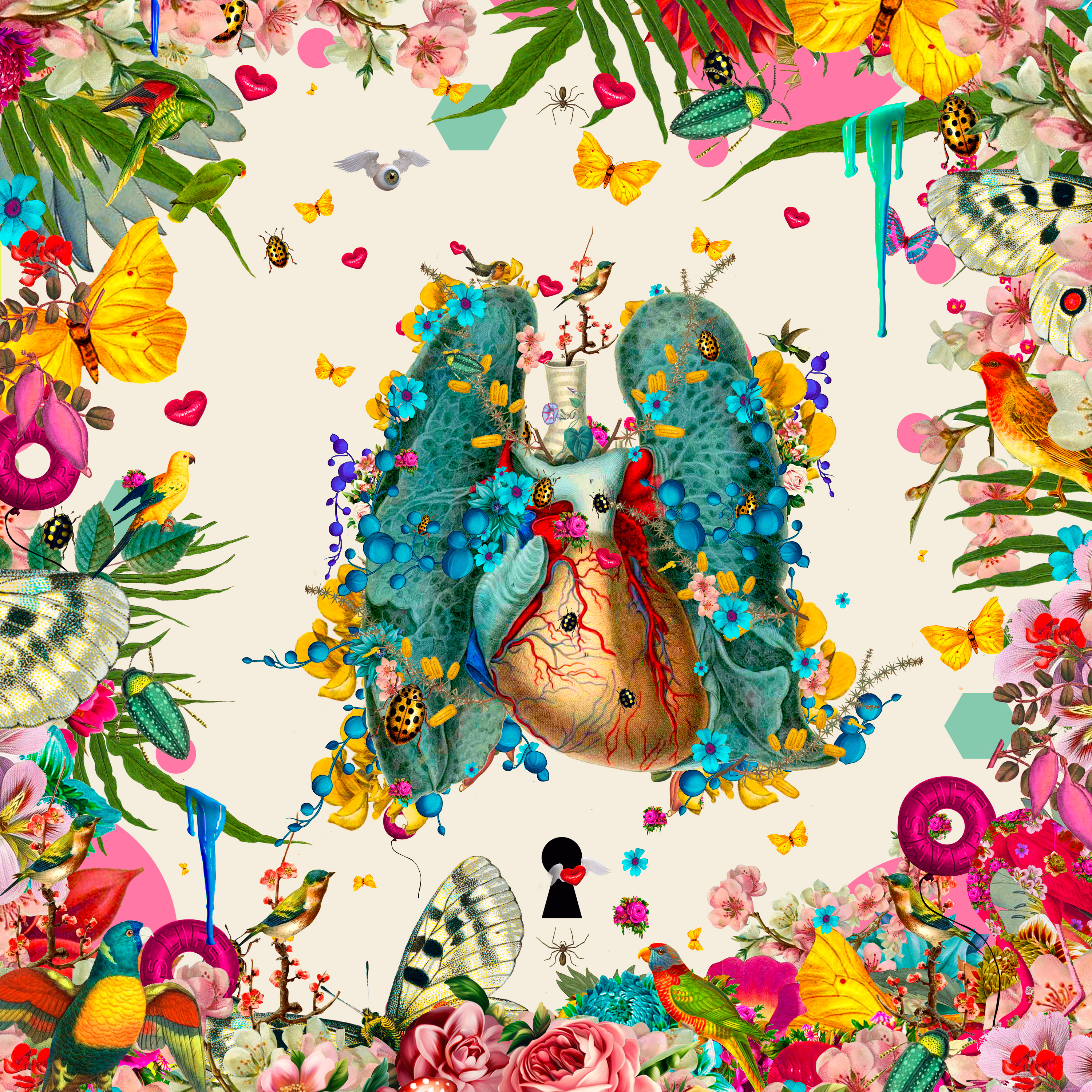The image is a vibrant and detailed art piece that appears to be an abstract, cartoonish portrayal of human organs, specifically the heart and lungs. These organs, which are the focal point of the square image, are decorated and intertwined with a plethora of vivid flowers, leaves, and vines. The heart, situated at the very center, is surrounded by green lungs that are similarly adorned with floral elements. 

Throughout the image, there are small birds, including a yellow bird on the left and a yellow and red bird on the right, along with a little green bird on the left. There are also multiple butterflies, predominantly yellow, scattered around. Additionally, an eyeball with wings and heart-shaped leaves add to the whimsical nature of the piece.

The entire border of the image is densely packed with colorful vegetation, flowers, birds, insects, and heart shapes, creating a lively and nature-infused aesthetic. Notably, a keyhole with a heart at the bottom center and a black spider approaching it provide unique focal points. The overall impression is a bright, positive, and hippie-like tapestry of natural elements beautifully integrated with human anatomy.